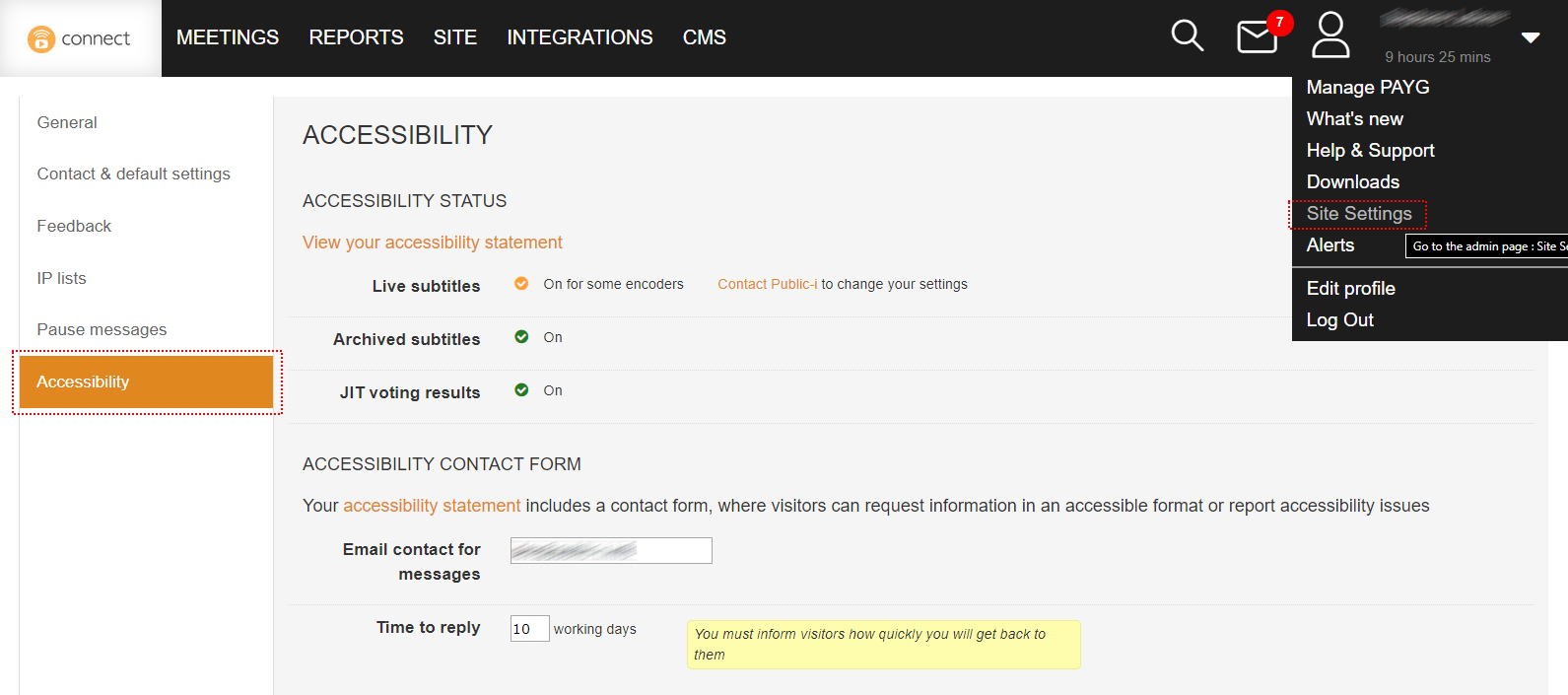A detailed screenshot of the "Connect" interface is displayed, prominently featuring an orange circle with a play button centered within it. The heading "Connect" is clearly visible, and beneath it, in white text on a black background, are the categories: "Meetings," "Reports," "Site Integrations," and "CMS." In the top right corner, there are icons for search, mail, and user profile.

The screenshot shows a notification stating "9 hours and 25 minutes," beside which the user's name is blurred out for privacy. A downward arrow indicates additional options, revealing: "Manage," "Page E," "What's New," "Help and Support," "Downloads," and currently highlighted, "Site Settings and Alerts."

Expanding further into "Site Settings," the highlighted sections include categories such as "General," "Contact and Default Settings," "Feedback," "IP Lists," "Pause Messages," and "Accessibility." Focusing on the "Accessibility" settings, it outlines several features:
- Accessibility status
- Viewing and modifying the accessibility statement
- Enabling live subtitles for certain encoders
- Providing an accessibility contact form that visitors can use to request accessible information or report issues.

Additionally, there's an "Email Contact for Messages" area, which is blurred out, with a clear response time mentioned: "10 working days." A yellow box underscores the importance of informing visitors about the response time.

Overall, the image captures intricate details of the "Connect" platform’s interface, highlighting its user-friendly navigation and emphasis on accessibility.